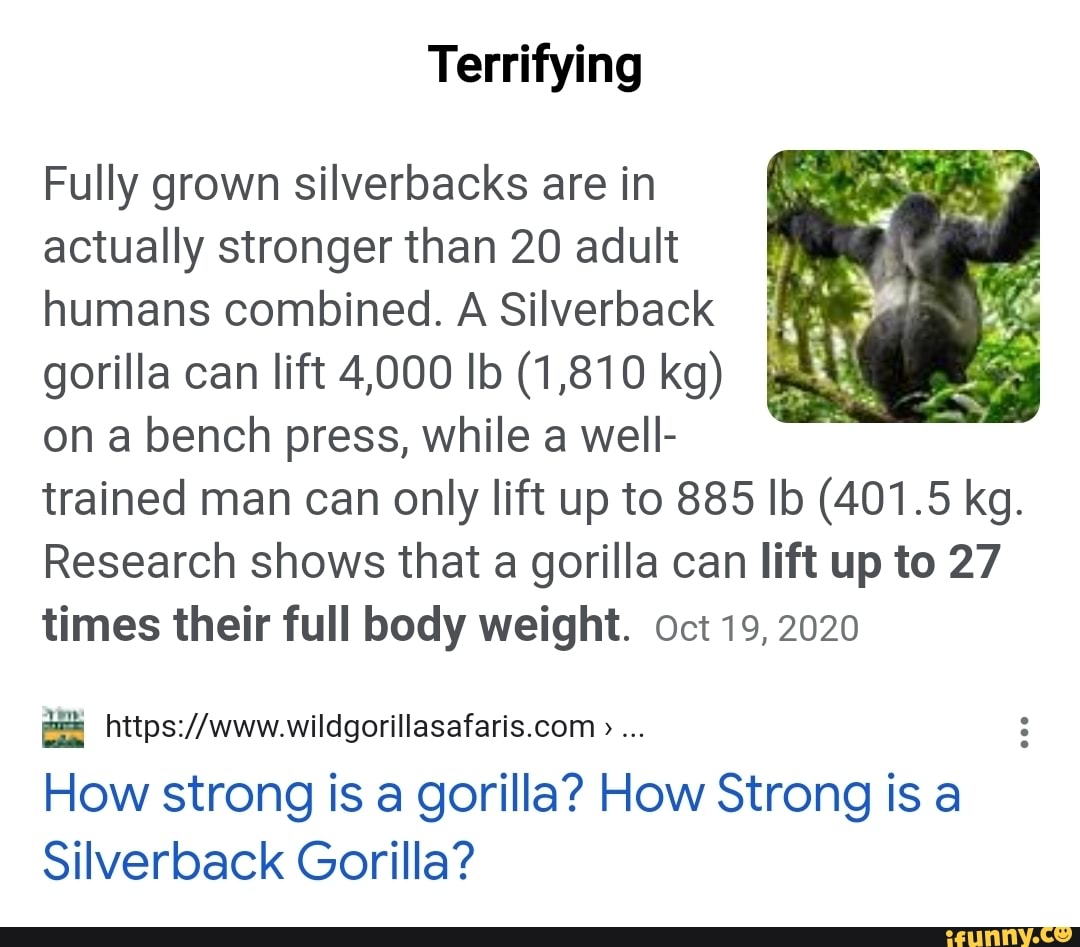The image displays a Google search snippet with an informative paragraph accompanied by a photo. The photo is set against a white background with the word "terrifying" written in black at the top, likely added by a user for humorous effect. The paragraph text is in a light gray-black font and reads: “Fully grown silverbacks are actually stronger than 20 adult humans combined. A silverback gorilla can lift 4,000 pounds on a bench press while a well-trained man can only lift up to 885 pounds. Research shows that a gorilla can lift up to 27 times their full body weight.” The paragraph is dated October 19th, 2020. Below the paragraph, there is an icon representing the website, and to its right, the URL www.wildgorillasafari.com is displayed. Underneath the URL, the page title "How Strong is a Gorilla? How Strong is a Silverback Gorilla?" is shown in prominent blue hyperlink text.